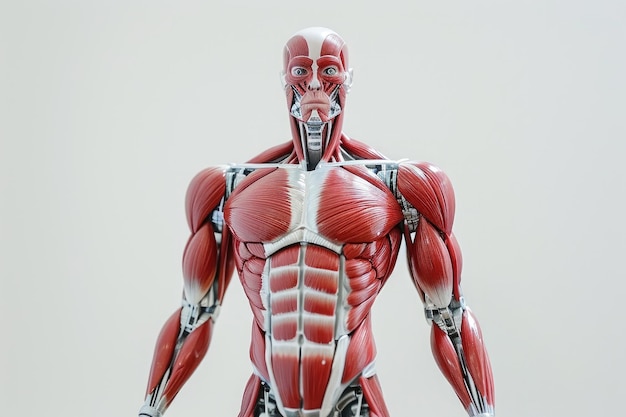This is a detailed photograph of a highly detailed model of the human muscular system, commonly used in advanced medical or science courses. The model is life-like and includes the head with visible eyes and frowning lips, devoid of skin to showcase the muscle tissue and fascia. The muscular structure is red, while the metallic elements, representing bones, are white. These metal parts articulate at the elbows and shoulder blades, and parts of the muscles can be removed to reveal deeper structures. The image captures the body from the hips up, with hands not visible. The background is an off-white, almost gray color, providing stark contrast to the red muscles. This detailed anatomical representation is intriguing and educational for those studying human anatomy.